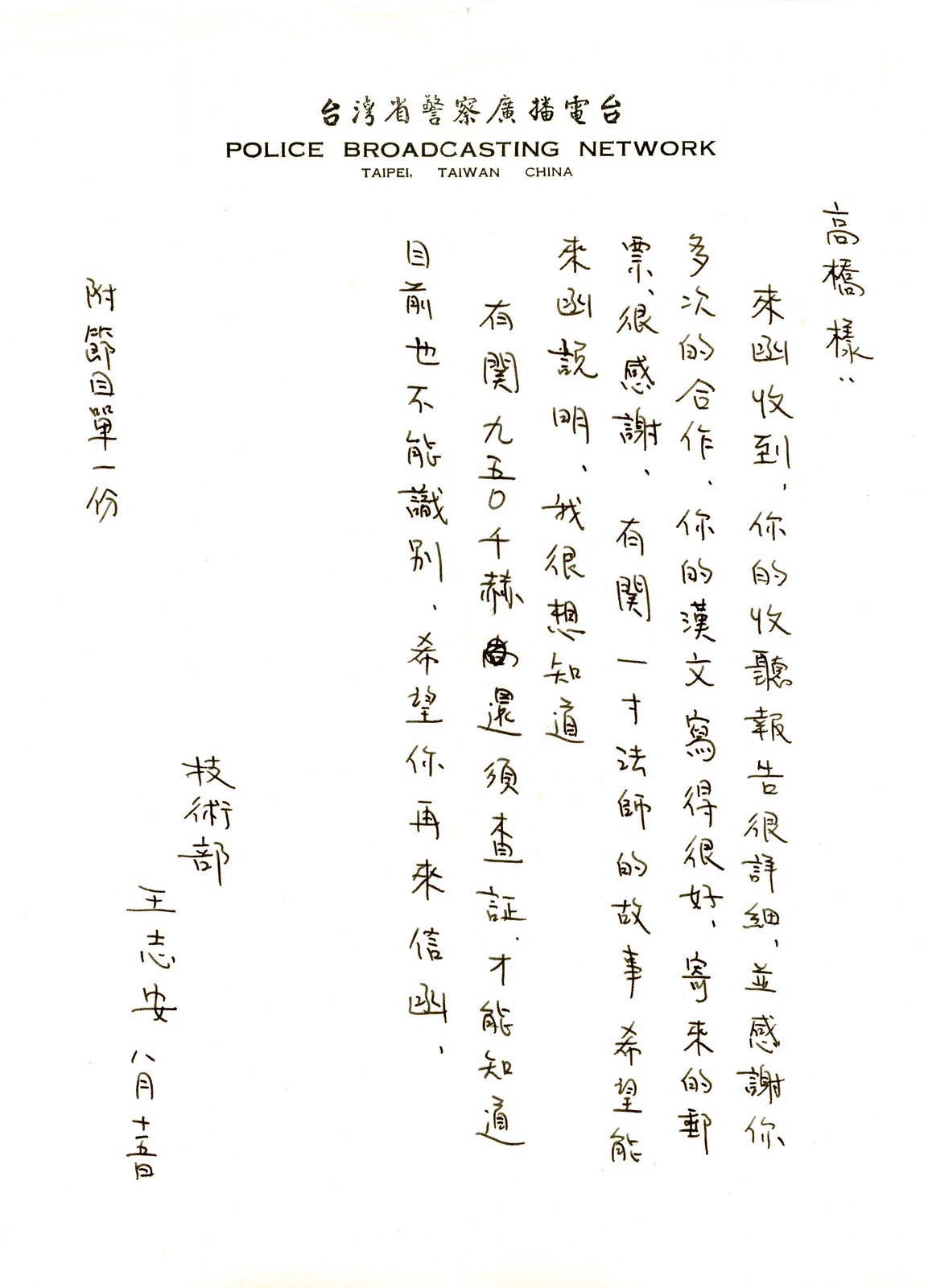The image is a sign or poster primarily featuring a solid white background with some text. At the top of the image in large letters, it reads "Police Broadcasting Network," followed by smaller text below stating "Taipei, Taiwan, China." The text at the top is written in both Chinese and English. The rest of the image is filled with columns of Chinese characters, which appear to be handwritten, resembling a correspondence or letter. The colors used in the image are predominantly white, black, and a hint of yellow. The overall style and setting suggest that it might be a promotional or informational poster for a radio station based in Asia.